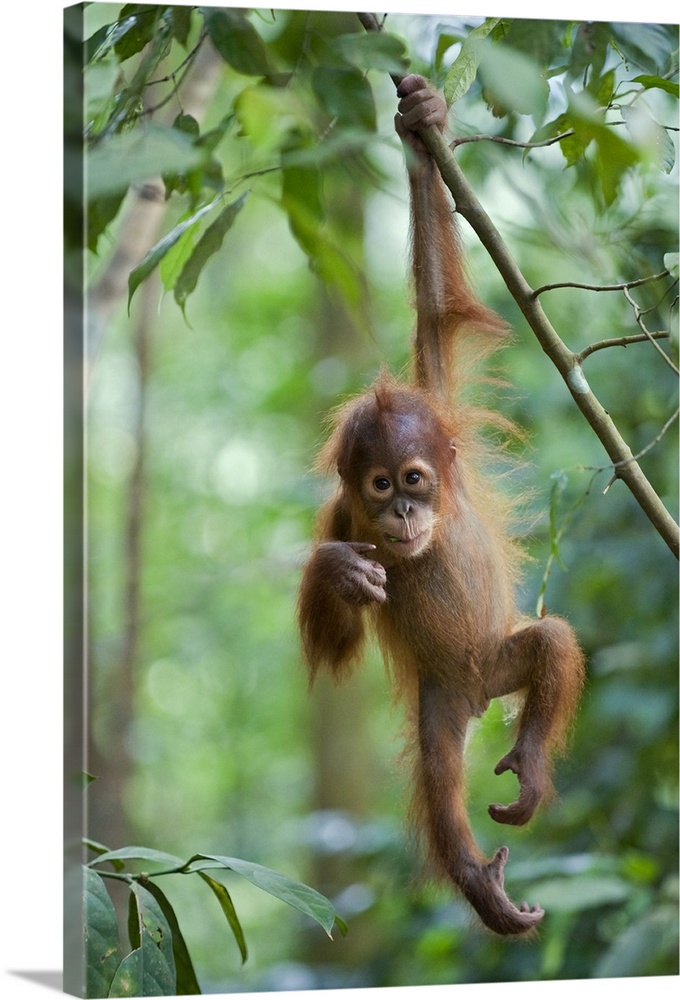In this detailed portrait, we observe a baby orangutan captured in a highly realistic photograph, possibly printed on a smooth, canvas-like surface. The young orangutan, with sparse tufts of ginger hair and noticeable bald spots, dangles from a slender tree branch with its left hand fully extended upward. The animal’s right hand is poised near its mouth, as if it may be eating a leaf, while its left leg bends at the knee and its right leg hangs freely. The orangutan’s expressive black eyes peer directly at the viewer, standing out against the lighter, whiter coloration of its chin and mouth area. The surrounding environment is lush with green leaves, some of which are sharply in focus, particularly at the bottom left of the image, while others form a blurred, leafy backdrop, emphasizing the main focus on the baby orangutan in the foreground.